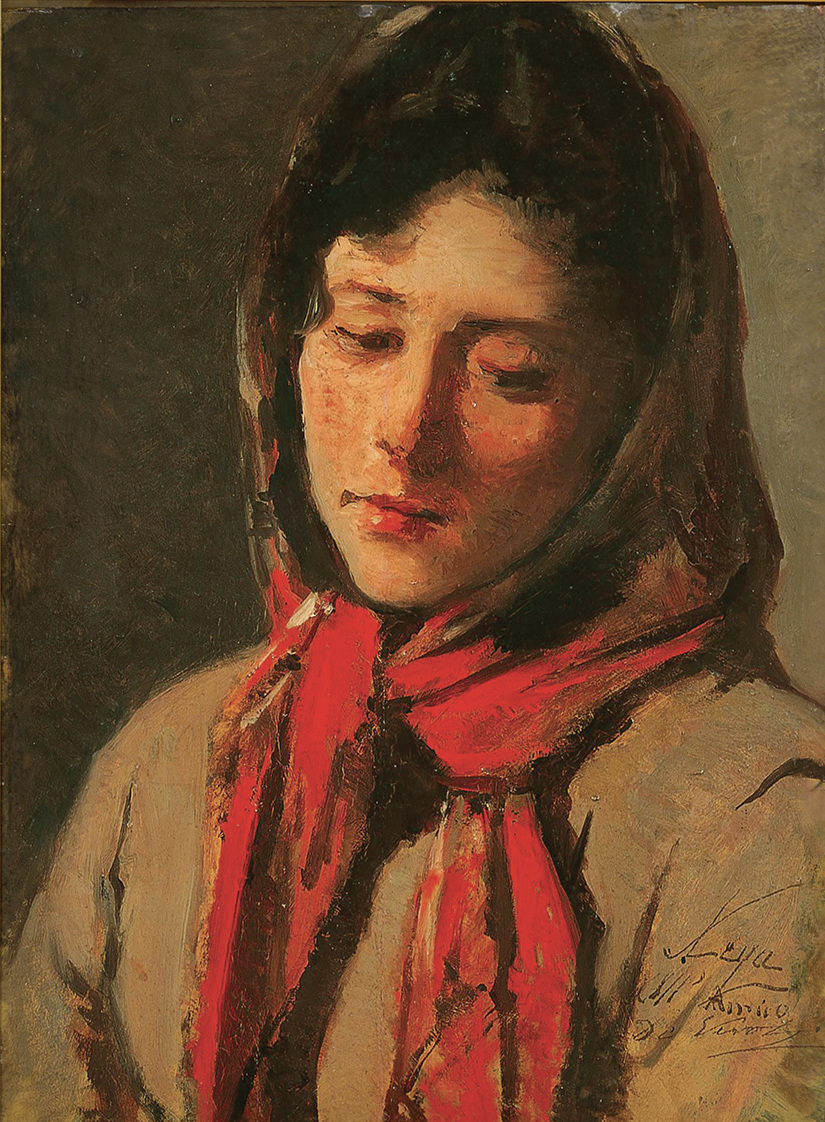This painting vividly portrays a woman in her 20s, exuding a palpable sense of sadness and contemplation. She has black hair with bangs, partially covered by a distinctive scarf. The scarf starts as a brownish hue on top of her head, transitioning into a vibrant red where it's tied around her neck, complementing her reddish lips. Her pale complexion is slightly blushed, enhancing the forlorn expression as her eyes look down to the left, avoiding the viewer's gaze.

The woman is adorned in a brown jacket, blending seamlessly with the subtly dark brown background. Her attire, a brownish-gray outfit, further merges her into the scenery, creating a cohesive, muted palette. The darker tones of the background intensify the emotional gravity of the piece, while her red scarf and lips stand out as the focal points amidst the muted colors.

Her posture and the composition — captured from her chest up with her head tilted slightly to the right — convey a deep sense of melancholy and wistfulness. The background, shifting from dark to lighter shades, perhaps mirrors her internal emotional landscape, adding depth to the overall poignant atmosphere of the painting. The gradient hues in the background range from olive green to varying shades of brown, encapsulating her in a somber and introspective ambiance.